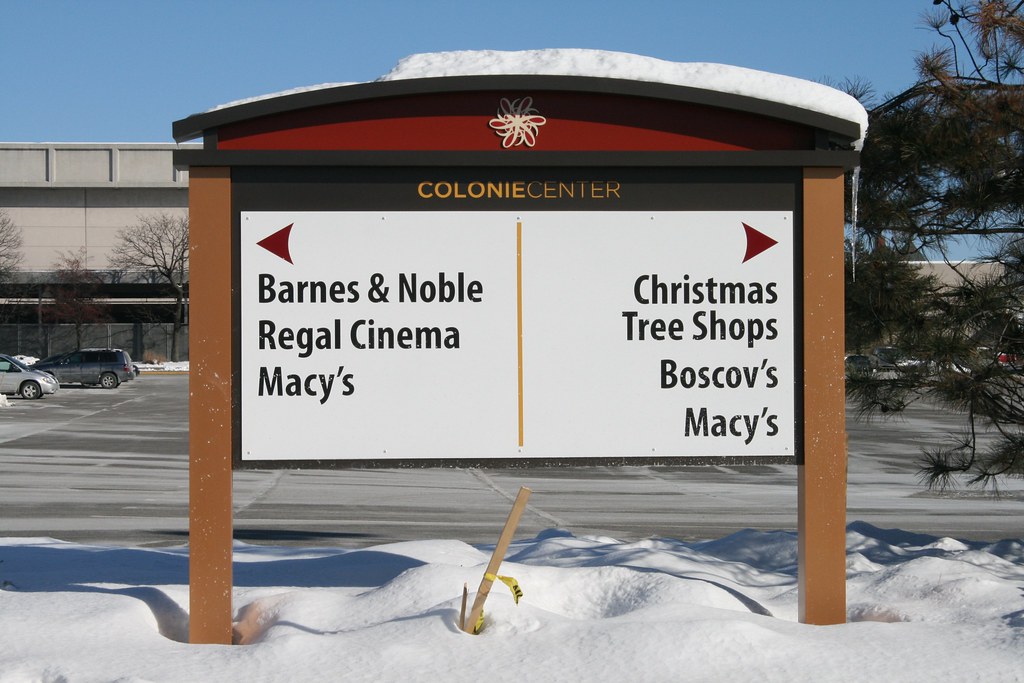This photograph captures an ornate sign positioned outside a mall during a snowy day. The sign is supported by two brown poles on either side and is topped with a red arch featuring a floral design at its center. Below the arch, the main sign is divided into two sections by a gold line. The top section includes a black horizontal bar with the text "Colony Center" in gray. On the left side of the sign, an arrow points left, indicating the direction of Barnes & Noble, Regal Cinema, and Macy's. On the right, another list with an arrow pointing in the opposite direction mentions Christmas Tree Shops, Boscov's, and Macy's once more. 

The sign and the surrounding ground are covered with a light dusting of snow, and an icicle hangs from the right side of the sign. Behind the sign, a nearly empty parking lot can be seen, with only two cars parked on the left side. The entire scene is enveloped in a gentle snowfall, adding to the serene winter atmosphere.